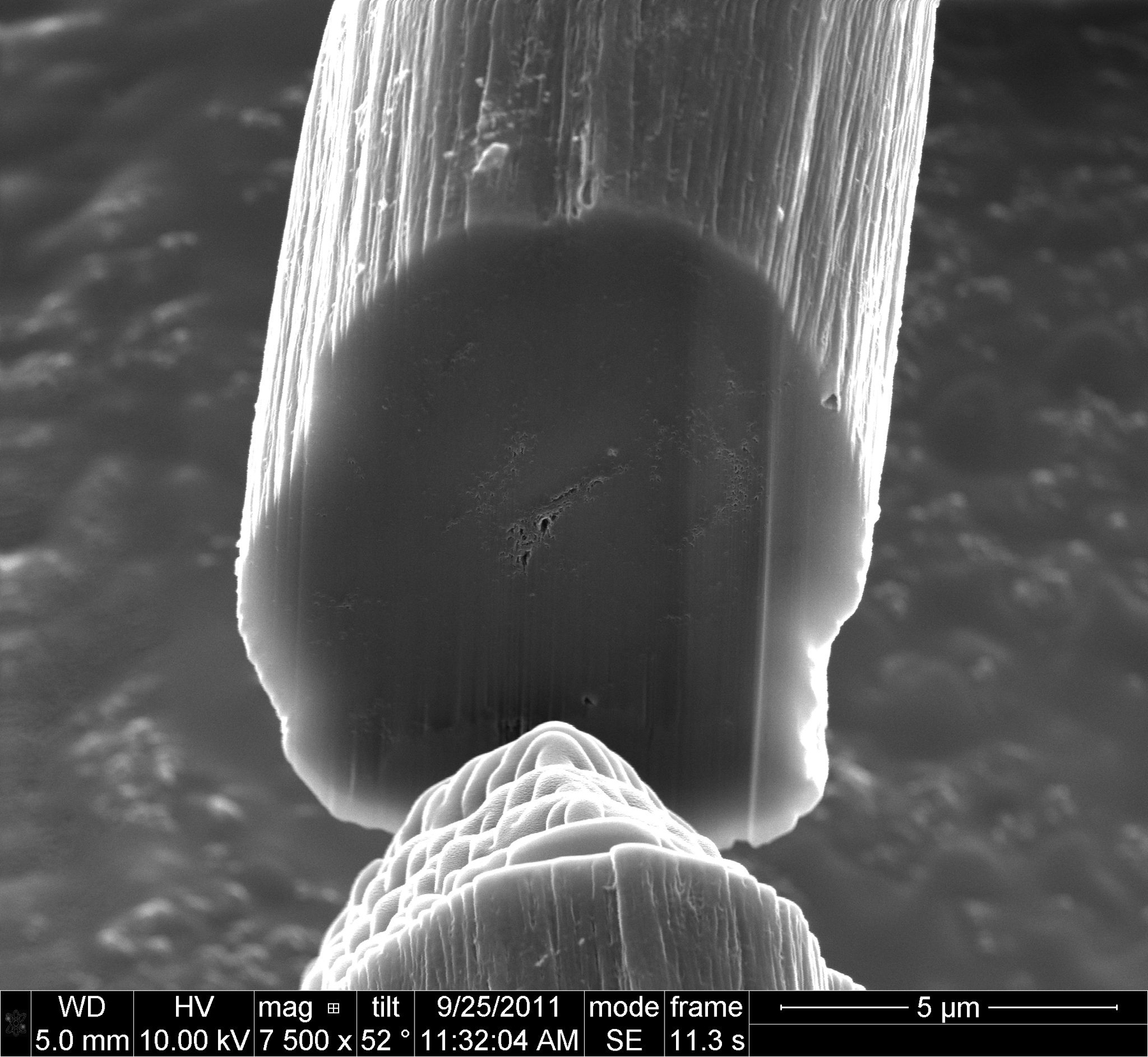The image appears to be a detailed microscopic, black-and-white representation, likely utilizing X-ray technology. Central to the image is a cylindrical column rising from the bottom, with a broken segment. This column, striated with crystallized lines, extends to the top of the frame, and is flanked by amorphous, dark-gray blobs. Below the main structure lies a formation resembling a mountain or petrified wood, depicted in various shades of gray. The background consists of a gradient gray sky with white cloud-like patterns. At the bottom of the image is a black strip displaying detailed annotations in white text: "WD 5.0 mm," "HV 10.00 kV," "MAG 7,500x," "Tilt 52°," "'9/25/2011," "11:32:04 AM," "Mode: SE," and "Frame: 11.3 seconds," along with "5 µm" on the bottom right.